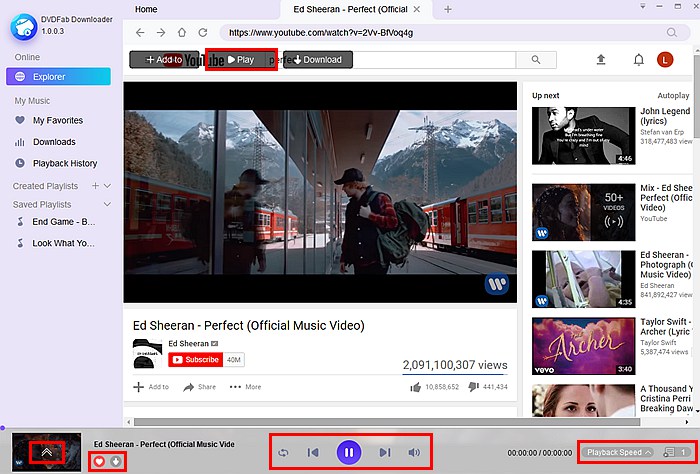The detailed screenshot features the DVDFab Downloader interface, showcasing two open tabs labeled "Home" and "Ed Sheeran - Perfect (Official Music Video)." The left pane includes a comprehensive menu with options such as "Online Explorer," "My Music," "My Favorites," "Downloads," "Playback History," "Created Playlists," "Saved Playlists," "In-Game," and more. Among the available playlists are "B..." and "Look What You...", possibly "U.S.Y.O...". 

Highlighted prominently is the main "Play" button enclosed within a red rectangle. A profile circle featuring the letter "L" is visible, suggesting a user profile or account. The highlighted video for Ed Sheeran's "Perfect" shows a scene with a man looking towards a building with a train passing behind him. This video is noted to have garnered an impressive 2,091,100,307 views.

At the bottom of the interface, several control buttons are displayed, including options for refresh, navigation arrows to the left and right, a speaker icon, and a pause button, providing ample functionality for media control.